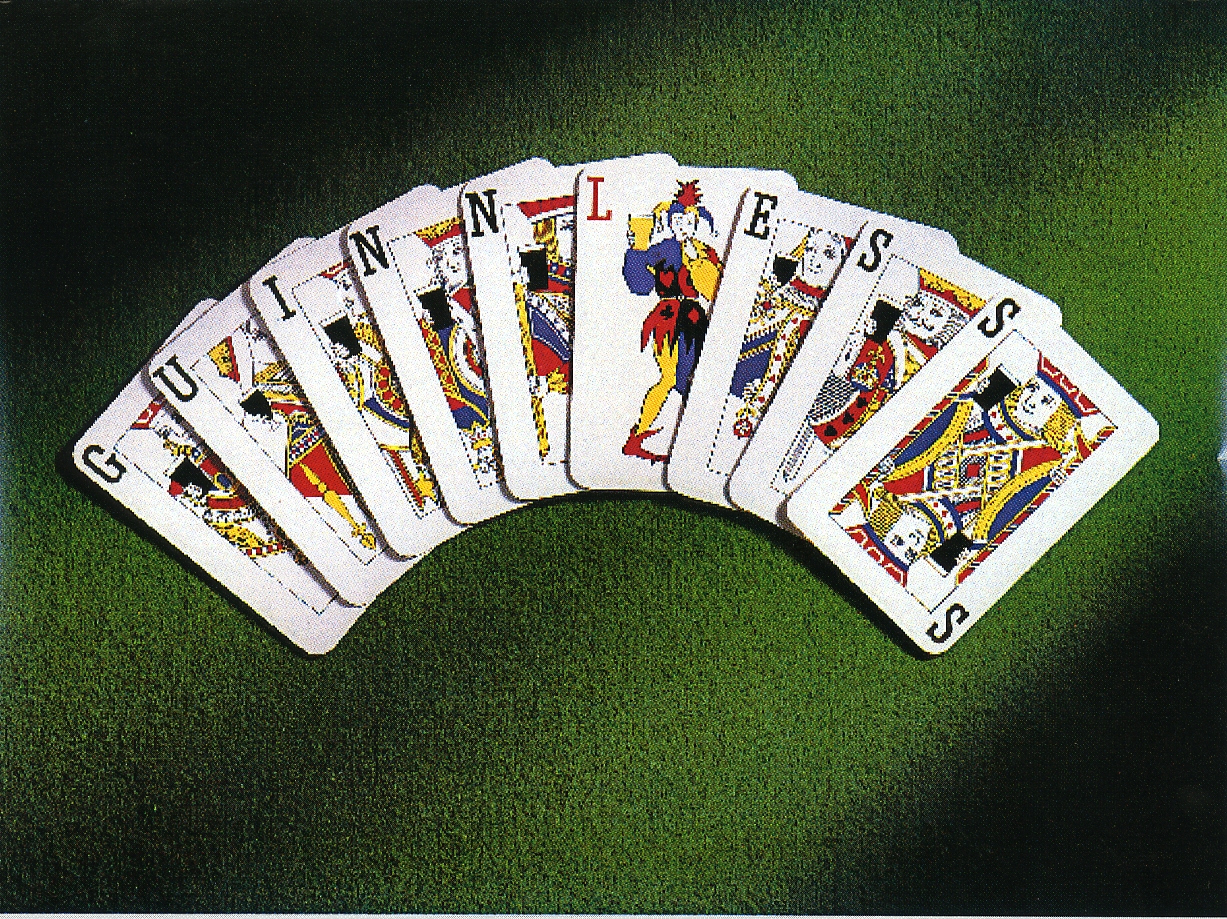A grainy photograph depicts white playing cards fanned out, face-up, across a green textured background, reminiscent of a felt poker table. The image is notably darker in the top left and bottom corners, with a slight shadow cast on the top right. Each card features a letter, seemingly arranged to spell "Guin-less" instead of "Guinness." From left to right, the sequence reads G-U-I-N-N-L-E-S-S: a Jack of Spades with a 'G', a Queen of Hearts with a 'U', a King of Clubs with an 'I', a King of Diamonds with an 'N', a Jack of Hearts with an 'N', a Joker with a red 'L', a Queen of Clubs with an 'E', a King of Spades with an 'S', and a Jack of Diamonds with an 'S'. The cards are carefully fanned out in the center of the photograph. The arrangement starts with the card on the far left lying beneath the others at an angle, and the fan culminates to the right, with each card slightly overlapping the previous one, creating a visually intriguing pattern.